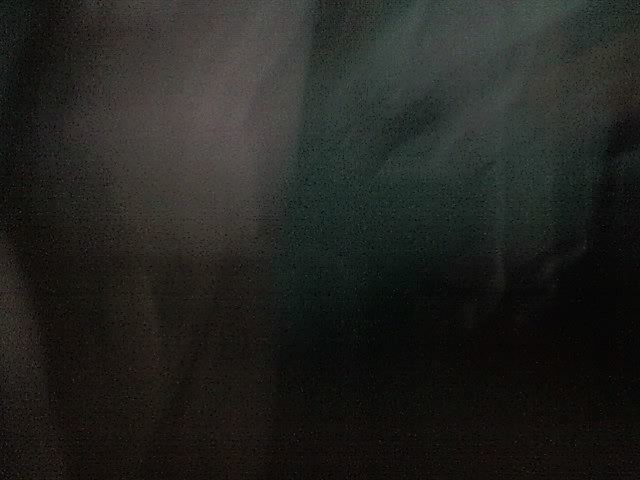This image presents an abstract, blurry composition, with distinct color segmentation across its quadrants. The upper right quadrant is dominated by a very dark bluish-green hue, while the lower right quadrant transitions into a deep, almost blackened, dark brown shade. This dark brown intensifies near the base, gradually blending into a dense forest green. The lower left quadrant exhibits a dark brown color that fades into a lighter brown towards the top, giving off a smoky appearance. Despite its indistinct forms, the image evokes a sense of abstract art, characterized by its well-defined, yet blurred, color partitions.